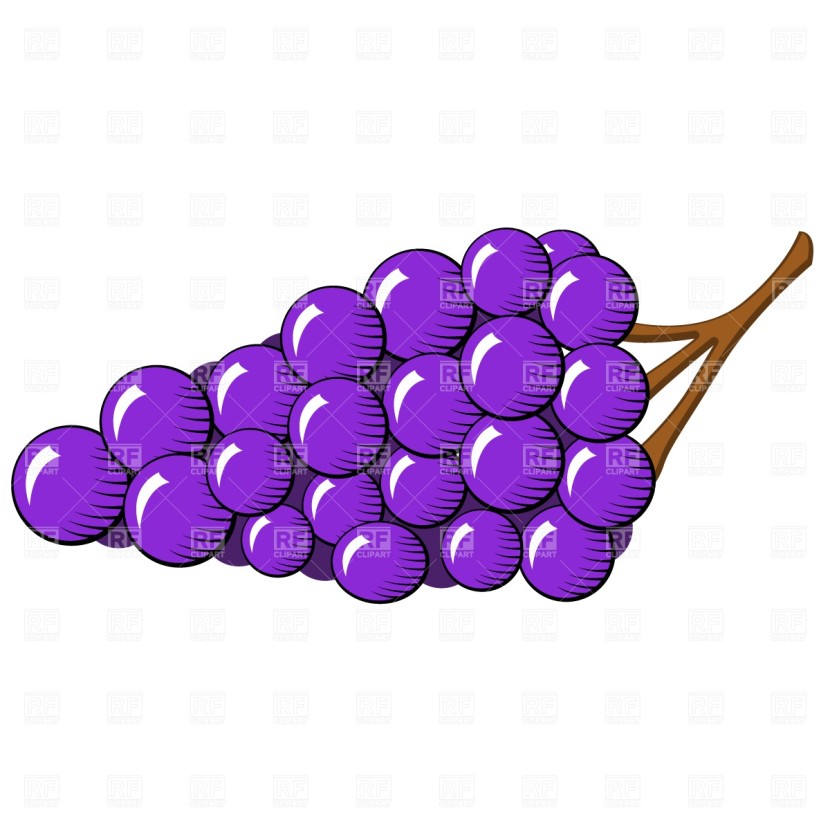This image depicts a vibrant illustration of a bunch of approximately 20 perfectly round, purple grapes, clustered together and attached to a light brown stem with dark highlights. Each grape features a white highlight to indicate where the light hits, emphasizing their glossy appearance. The illustration is designed in a distinctive, non-realistic style, typical of clipart. The entire bunch appears to float against a completely transparent background, adding to its clipart feel. Overlapping across the image and on each grape is a rectangular purple watermark with the letters "RF" in darker purple, and smaller, illegible text below, suggesting a tag for royalty-free clipart.